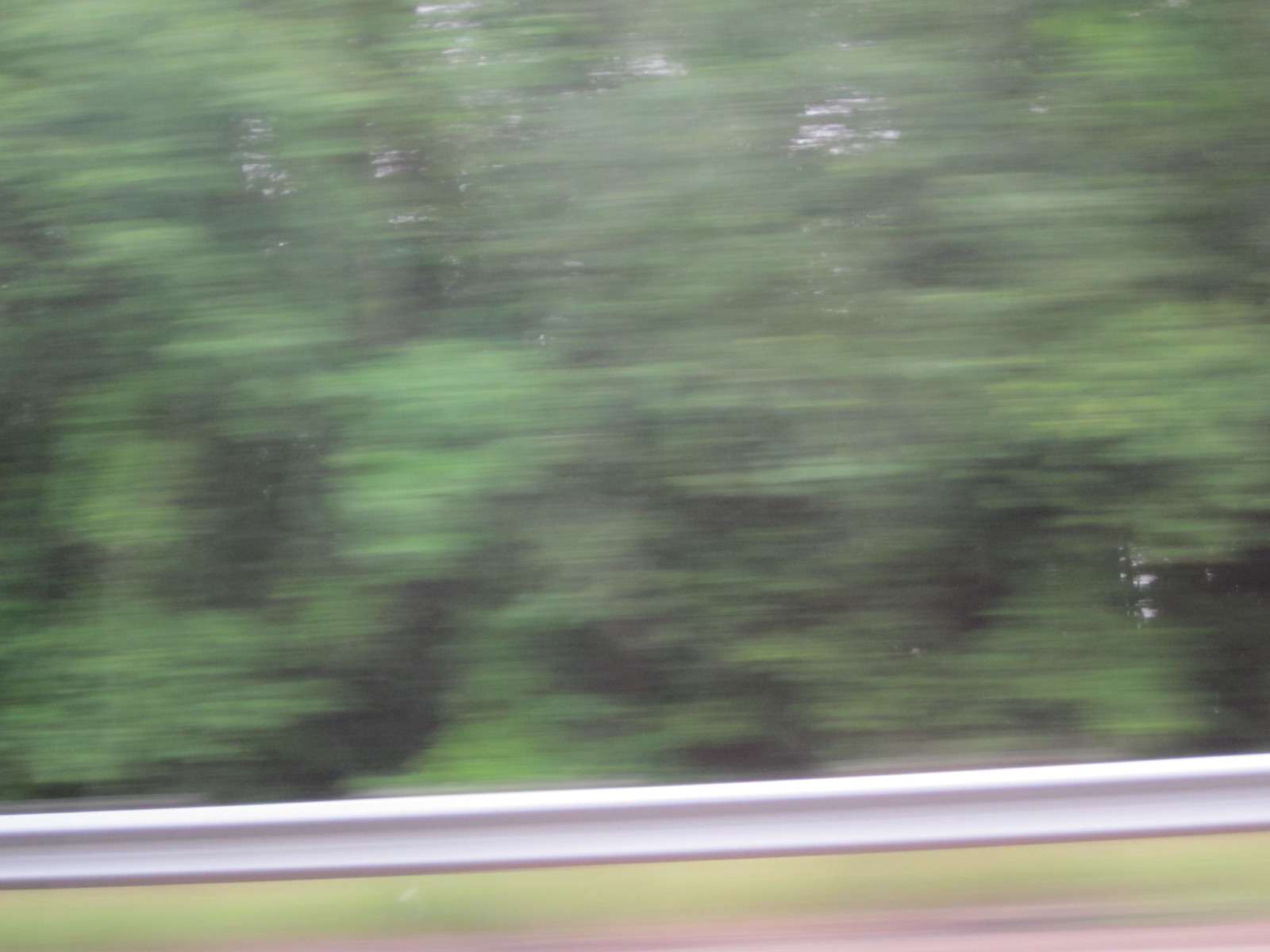A blurred photograph captures the rush of motion outside a vehicle, possibly a speeding car or train. The scene is viewed through a window, identifiable by a white, wooden frame at the bottom and a surrounding green frame. Outside, the scenery flies by, predominantly featuring a dense forest of trees. The rapid movement renders the trees as streaks of light and dark green, interspersed with occasional gaps that reveal glimpses of the sky. The overall effect is a testament to the speed and transient nature of travel through lush woodland.